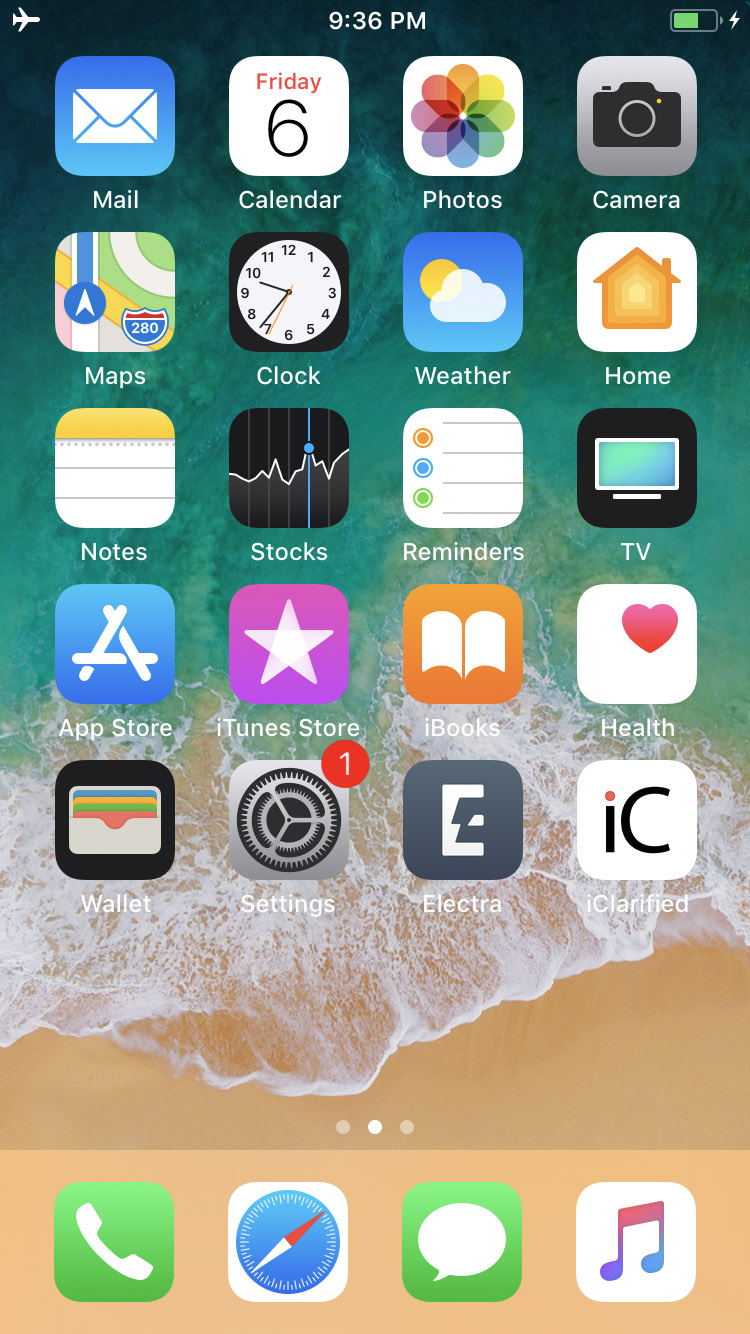Screenshot of a classic Apple mobile layout, most likely from an iPhone or iPod Touch. The time displayed at the top is 9:36 PM, with the battery approximately 70% charged. The layout features the standard four-icon rows typical of Apple devices. 

The top row includes icons for Mail, Calendar, Photos, and Camera. The second row shows Maps, Clock, Weather, and Home. Following those, the third row contains icons for Notes, Stocks, Reminders, and TV. The fourth row has the App Store, iTunes Store, iBooks, and Health, followed by Wallet, Settings, and Electra. 

There is a blank row before the dock, which is situated at the bottom of the screen. The dock includes four main icons: Phone, Safari, Messages, and Music. This screenshot is from the second of three pages of apps on the device.